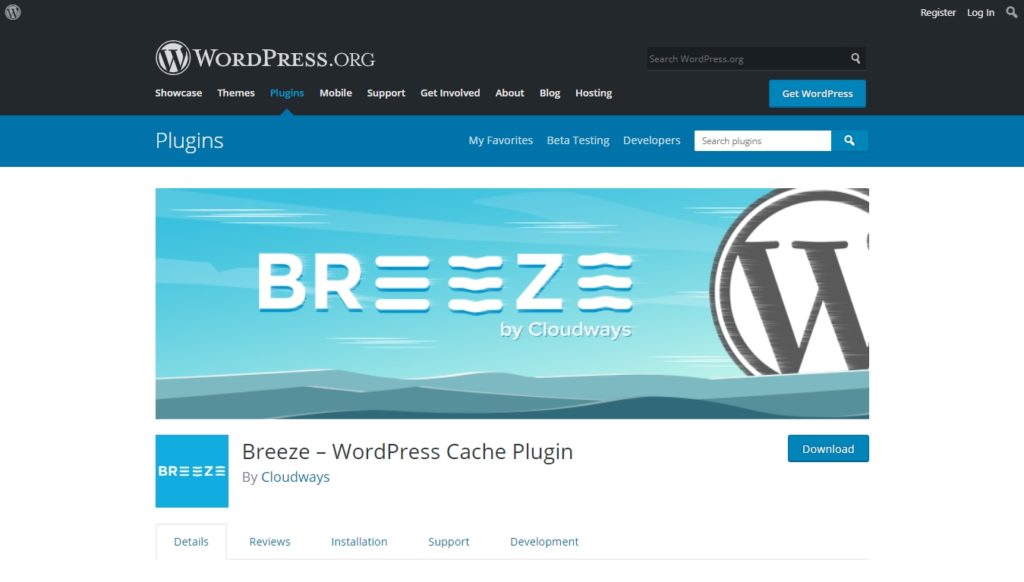The image depicts a webpage from WordPress.org, specifically showcasing the Plugins section. At the top of the page is a navigation bar with various subcategories including Showcase, Themes, Plugins (which is currently selected), Mobile, Support, Get Involved, About, Blog, and Hosting. Adjacent to the "Plugins" category are additional options labeled My Favorites, Beta Testing, and Developers. 

To the right, there is a search bar labeled "Search Plugins" for easy plugin discovery. Below the navigation bar, a large banner prominently features the "Breeze by Cloudways" plugin. The word "Breeze" is styled uniquely with the letter 'E' replaced by three horizontal waves. Next to the plugin name is a prominent blue "Download" button. 

Directly beneath this banner, the Breeze logo is displayed again, along with the plugin's full name: "Breeze WordPress Cache Plugin by Cloudways." At the bottom of the banner, there are tabs for additional details about the plugin, including "Details," "Reviews," "Installation," "Support," and "Development," all rendered in black font on a black background with white text.